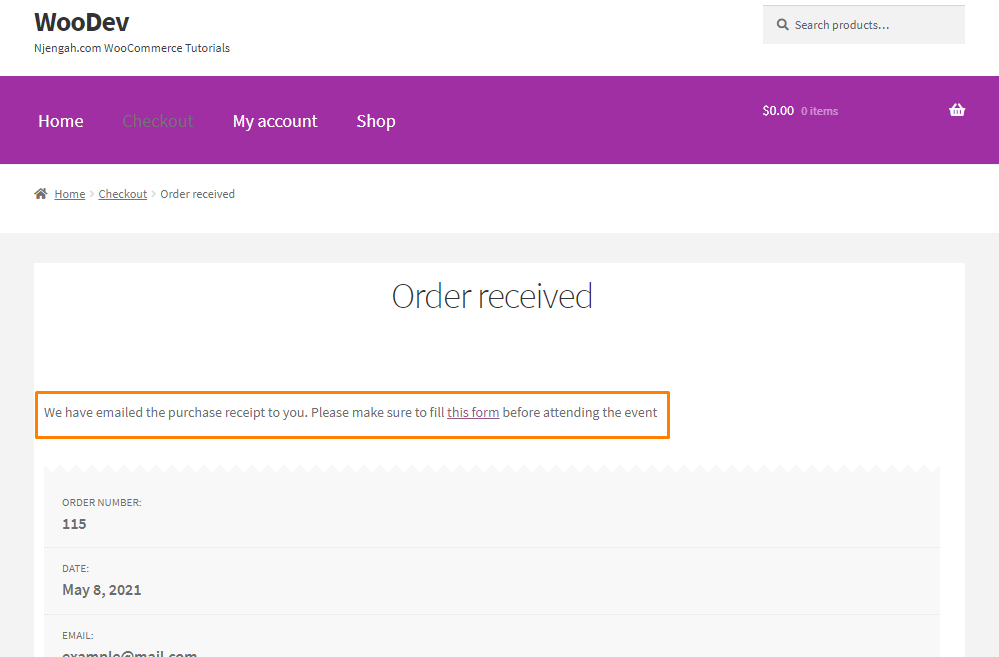The website features a clean, structured layout with distinct sections and a clear focus on user navigation. At the top, the site prominently displays its title "WooDev," with both the "W" and "D" capitalized and rendered in bold black letters. Directly beneath this title, the subtitle reads "Nginga.com Woo Commercial Tutorials."

On the right edge of the header is a search bar, accompanied by a magnifying glass icon, and labeled "Search Products." Just below the header is a striking purple navigation banner, which features several options in white text on the left: "Home," "My Account," and "Shop." These options are grouped alongside the "Checkout" option, which is displayed in gray. To the right side of this purple banner, the shopping cart is displayed, currently showing "0 items" and a total of "$0.00."

Centered below the banner in a section with a gray outline and a white background, the text "Order Received" is displayed in gray. Further down, a rectangular orange-outlined box contains the message: "We have emailed the purchase receipt to you. Please make sure to fill this form before attending the event."

The final details listed below this box include the order number, "Order Number: 115," the date, "Date: May 8, 2021," and the email address, "Email: example@gmail.com."